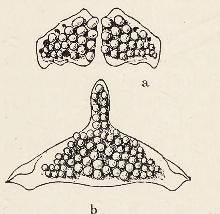The image features a detailed black-and-white drawing on a white background. It consists of three distinct sections. At the top, two smaller drawings are situated next to each other. The left drawing, labeled with a lowercase 'a,' depicts a circular shape with numerous small, round objects inside, resembling seeds or pebbles. The right drawing has a similar circular structure with the same small, round objects and is also labeled with a lowercase 'a.' Below these, a larger triangular shape resembling a cucumber sticking out from the ground houses the same round elements inside and is marked with a lowercase 'b.' The meticulously crafted diagram, though visually simple in its monochromatic presentation, intricately details these shapes and their consistent internal elements.